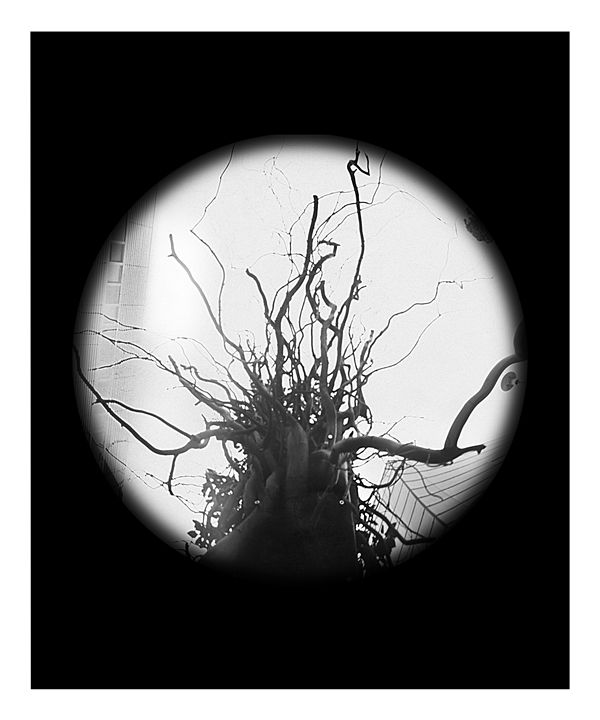This black-and-white photograph, presented in portrait orientation, features a striking dark background punctuated by a prominent white circle in the center. Within this circle lies a detailed depiction of a leafless tree, characterized by its numerous scraggly branches extending in various directions. The limbs of the tree are particularly dense at the bottom, gradually dispersing towards the top and sides, creating a visually complex root-like structure. To the left of the tree, part of a high-rise building is visible, its outline softened and slightly out of focus. On the lower right side of the circle, another building with a mirrored surface and a multi-floored, glass design appears, adding depth and a touch of modernity to the scene. A feathered edge around the circular image lends a soft silhouette effect, blending the stark contrast between the black background and the vivid white circle, and enhancing the overall enigmatic atmosphere of the photograph.